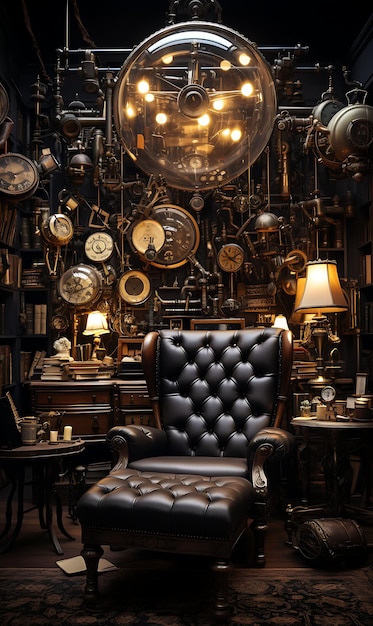In this image, a dark, busy room with an eerie feeling is captured. The focal point is a blackish-brown leather sofa adorned with an ornament, positioned on a multi-toned brown and black rug. To the side of the sofa, there is a coffee table holding white candles and grey-brown pots. Behind this setup, an array of end tables and a desk cluttered with books, clocks, candles, and various objects can be spotted. The desk is particularly prominent, featuring drawers and a spread of books, adding to the cluttered atmosphere.

Dominating the background is an overwhelming multitude of clocks in various sizes, both small and large, adorning the walls. Above the sofa, a network of metal pipes weaves through the space. Suspended amidst these pipes and clocks is a clear plastic globe containing bright white and yellow lights, casting an eerie glow. The walls' color is obscured by this dense array of objects and fixtures, enhancing the room's dark, crowded aesthetic. Lamps scattered throughout the space provide additional illumination, emphasizing the numerous metallic pipes and tubular structures that contribute to the room's industrial, cluttered look.